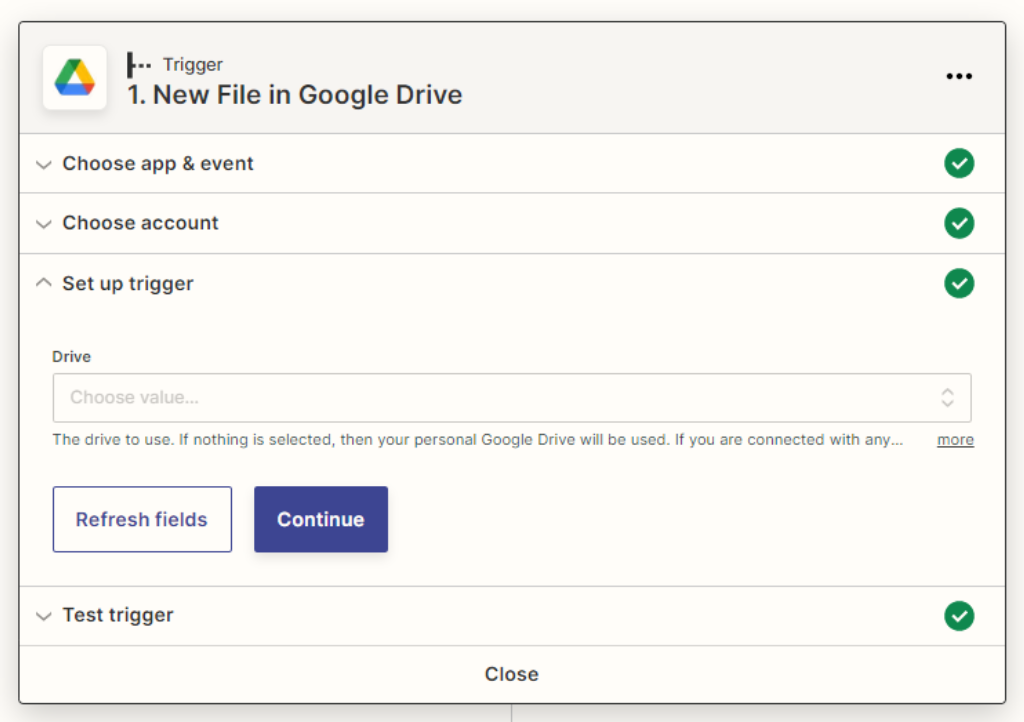The image appears to be a screenshot from a website, possibly related to setting up a Google Drive integration. In the upper left corner, there's a white square containing a colorful triangular Google Drive logo. To the right, the text reads "Trigger," followed by "New file in Google Drive." Below this, there's an option labeled "Choose app and event," which has a green circle with a check mark next to it. This is followed by "Choose account," also marked with a green circle and check mark, and "Set up trigger," which is similarly marked with another green circle and check mark.

Beneath this section lies a considerable blank space, followed by the word "Drive." Below "Drive," it says "Choose value," which seems to be a box where you can type or select an option. Further down, there's a rectangle outlined in blue that reads "Refresh fields," and to its right is a blue rectangle with white text stating "Continue." Finally, another line reads "Test trigger," with a green circle containing a check mark to the right. At the bottom center in black text, the word "Close" is displayed.